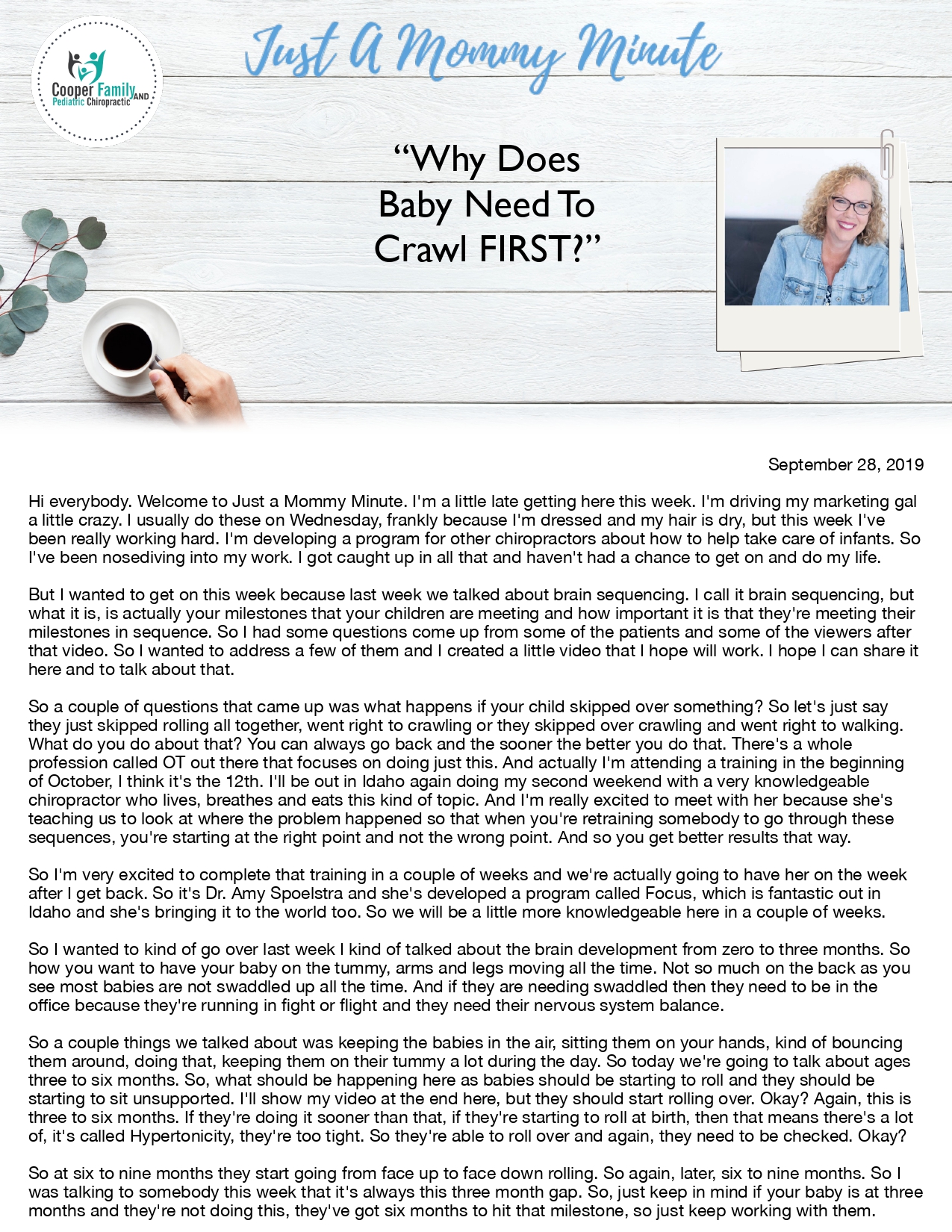Here is a detailed and cleaned-up caption for the image described:

---

The image is a screenshot of an article published on a website. The title, "Just a Mommy Minute," is prominently displayed at the top center, written in a bright blue cursive font. On the left side, there is a circular website icon featuring a simplistic representation of a family: two larger figures, one black and the other teal green, with a smaller green humanoid figure in the center. Below the icon, "Cooper Family" is written in black text.

The main article title is centered beneath the website icon, reading "Why Does Baby Need to Crawl First?" in black text with "FIRST" emphasized in all capital letters and quotation marks. Next to the article title is a decorative graphic of some green leaves on a brown stem, and below it, an image of a white ceramic saucer and cup, likely containing black coffee, held by a person's hand.

To the right of the article title is a square photograph of the author, outlined in black. She is a woman with medium-length curly brown or blonde hair, wearing black-rimmed glasses and smiling. She is dressed in a light blue denim shirt.

The article text, written in black on a white background, was published on September 8, 2019, indicated in small text on the right side. The article expands on the topic of why it is important for babies to crawl first.

---

This caption provides a detailed and organized description of the screenshot, highlighting key elements and their positions in the image.